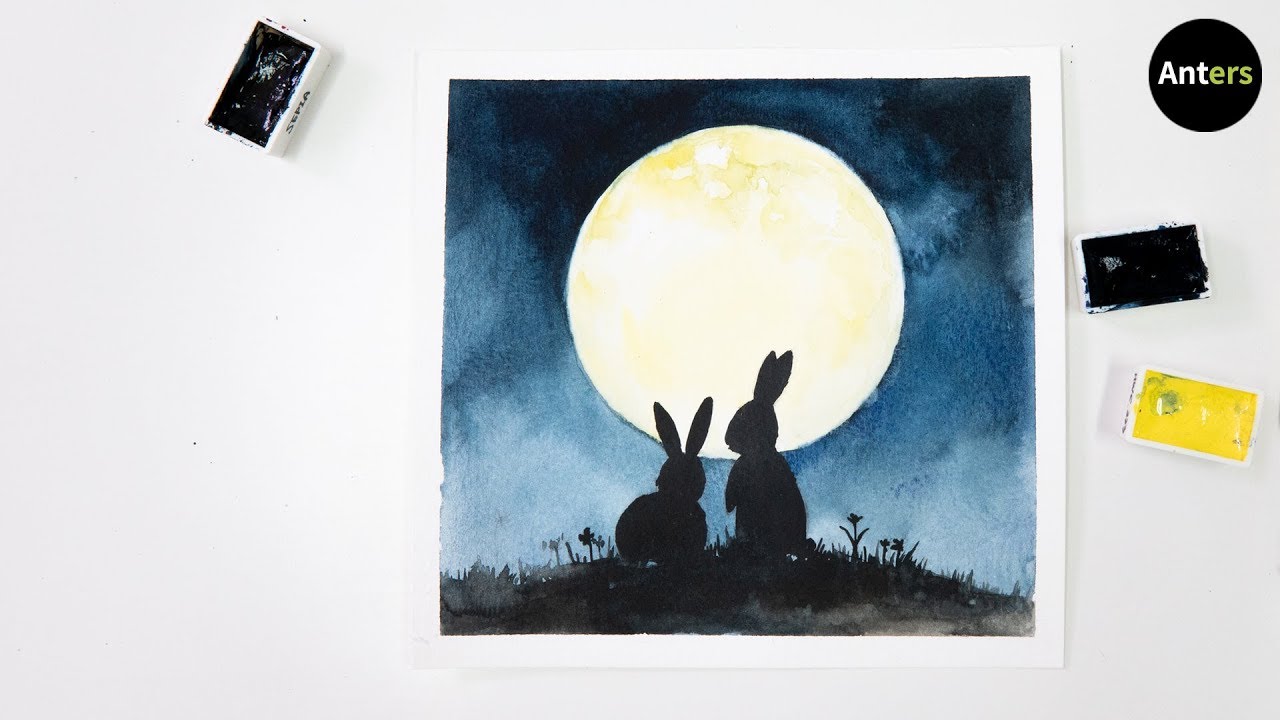The image presents an off-white rectangular canvas, centered by an intricately framed white square. This square houses a night scene dominated by a large, luminous light-yellow moon, which bathes the landscape in its glow. The background features a serene dusky night sky painted in shades of navy blue, black, white, and gray. At the forefront, atop a gently sloped knoll or hill, two rabbits sit together in silhouette, their ears attentively upright as they gaze at the moonlit scenery. The knoll is adorned with the delicate silhouettes of grass and blooming flowers, possibly dandelions, adding to the whimsy of the scene. To the left of the central picture within the off-white frame, a white container of black paint can be spotted, flanked on the right by containers of dark blue and yellow paint. In the upper right-hand corner, a logo bearing the word “ANTERS”—with “A-N-T” in white and “E-R-S” in green—adds a distinct touch. The painting, created with possible sponge-dabbing techniques, evokes a peaceful, romantic ambiance, depicting the rabbits in a tranquil moonlit moment.